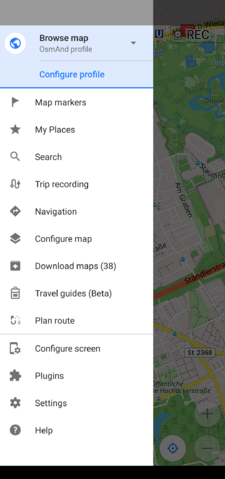This screenshot displays a detailed interface of a digital map application filled with various functionalities and settings. The background features the colorful map itself, showcasing geographic details in vibrant hues contrary to its monochrome mentions. In the foreground, an overlay menu is visible on the left side, offering multiple options such as 'Map Markers', 'My Places', and a search bar to facilitate navigation and trip planning. Additional functionalities include 'Trip Recording,' 'Navigation,' and 'Configure Map,' allowing users to tailor their map views and download additional maps; currently, it indicates 38 downloadable maps available. The menu also provides 'Travel Guides' and a 'Plan Route' feature to assist with itinerary creation. Below this section, another bar offers further options like 'Configure Screen,' 'Plugins,' 'Settings,' and 'Help,' ensuring comprehensive customization and user support.